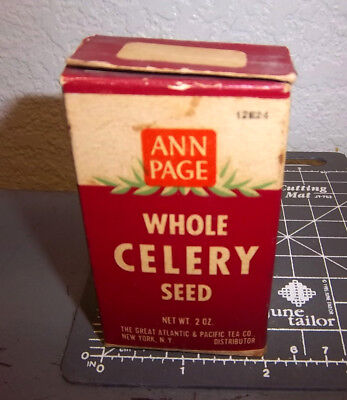In the image, we see a vintage cardboard box of whole celery seed, labeled "Ann Page." The box appears to be from the mid-20th century, possibly the 1950s to 1970s, and shows significant signs of aging and wear. The design features a burgundy-red upper half with a yellowing white strip and an orange square that prominently displays "Ann Page." Below this, green leaf stems trail out from the text. The lower half of the box is also burgundy-red with yellowish-white text that reads, "Whole Celery Seed," and indicates a net weight of two ounces. The box's edges and seams are chipping away, revealing its age. Additionally, it bears the name "The Great Atlantic and Pacific Tea Company, New York, New York."

The box is placed on a gray table, atop a plastic cutting mat that resembles a clipboard, used for measuring fabric lengths. This cutting mat has a white grid with measurement markings and the partially visible name "June Taylor." The condition of the box and the details on the mat suggest a historical and utilitarian domestic setting.